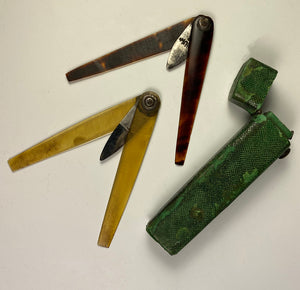The image features three main objects lying flat on a light gray background, taken from an overhead perspective. On the bottom right is a dark green rectangular case with paint peeling off, revealing lighter green patches. The case has a square cap on its upper right side, which is open and attached by a hinge. To the left of the case are two fold-out knives. The knife at the top has dark brown handles and a partially unfolded blade that is short and silver with black streaks. The bottom left knife has almost translucent yellow plastic handles, exposing the internal mechanisms. Its blade is silver in the middle, transitioning to black towards the tip, held together by a visible circular pivot. Soft shadows cast by the light accentuate the objects' details.